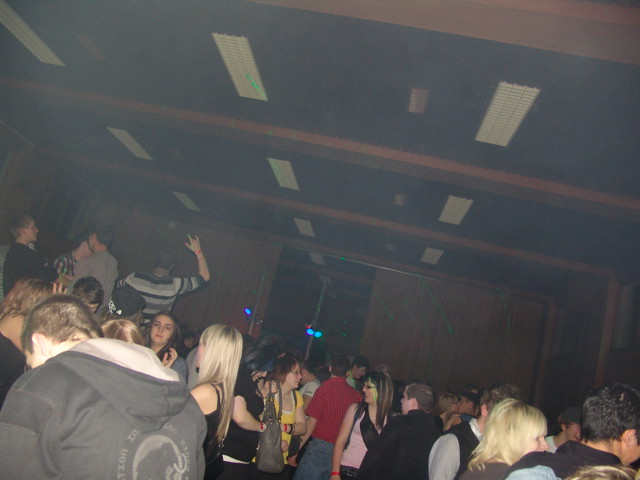In this indoor photo, a crowded room captures the lively essence of what appears to be a dance event or social gathering. The space is adorned with brown paneling on the walls, a ceiling comprised of brown beams interspersed with white vents, and a noticeable haziness, possibly due to smoke. The overall scene is bathed in a faint blue light that hints at a nightclub ambiance. The room is bustling with semi-casually dressed individuals, some with their hands raised, possibly dancing or gesturing.

In the foreground and middle of the image, attendees are engaged in animated conversations while others take to dancing. Notably, at a slightly elevated platform or stage area, people can be seen above the crowd, suggesting a level difference in the room's layout. On the left side of the image, a man in a gray jacket stands out, along with another man in a striped shirt making a gesture with his right hand near three men having a discussion.

Details such as the slanted angle of the photo and the visible ceiling lights enhance the dynamic and busy atmosphere of the scene. In the background, a door framed by blue lights opens up to another part of the venue, adding depth and an air of mystery to the festive setting.